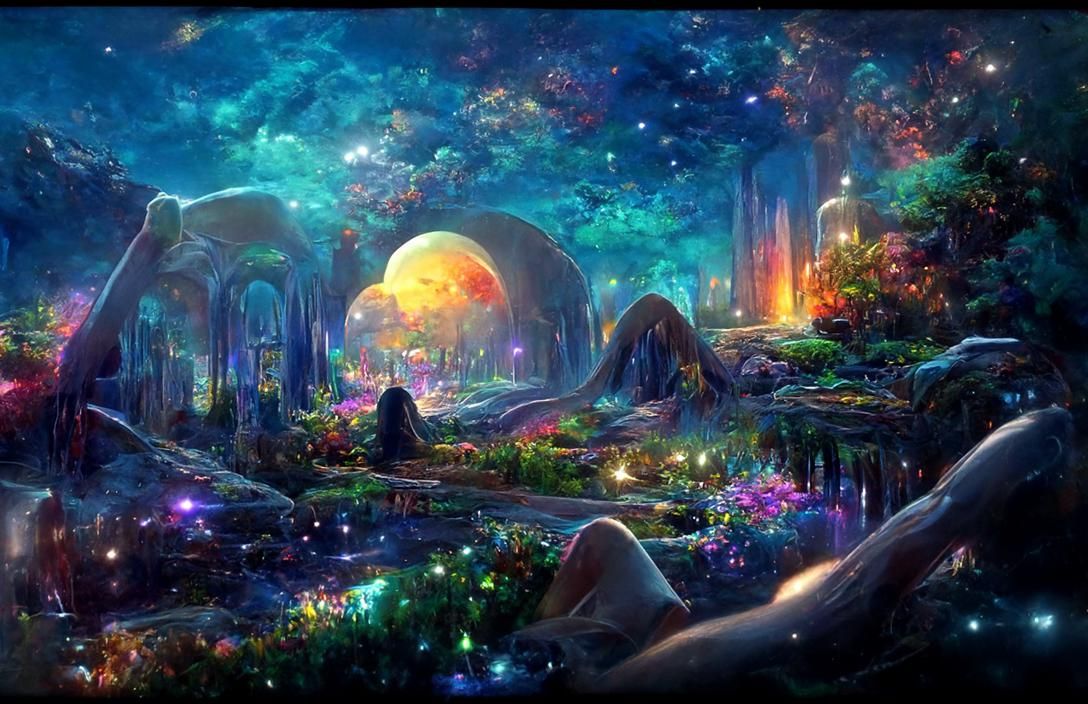The image is a fantastical painting depicting a magical nighttime forest scene. Neon blue clouds interspersed with iridescent colors of pink, yellow, and purple dominate the sky, setting a mystical tone. Glittering lights in similar hues dot the landscape, adding an otherworldly sparkle. The forest is replete with various plants in shades of green, red, and pink scattered throughout, enhancing the enchanted ambiance.

A serene stream winds through the forest, its surface reflecting the myriad of colors and lights surrounding it. Little will-o'-the-wisps float in the air, resembling stars against the dark backdrop. Natural formations like rounded geometric rocks rise impressively from the ground, while what appears to be the entrance of a cave or a naturalistic structure glows warmly with orange light, stalactites visible inside. Additional glowing orange highlights accentuate a potential rock outcrop or waterfall in the background.

Despite the night setting, the scene is alive with color and light, with purple and blue flowers illuminated by specks of yellow adding to the dreamlike quality. The overall style seamlessly blends elements of a magical forest with striking, vibrant details, inviting viewers into this enchanting, otherworldly realm.